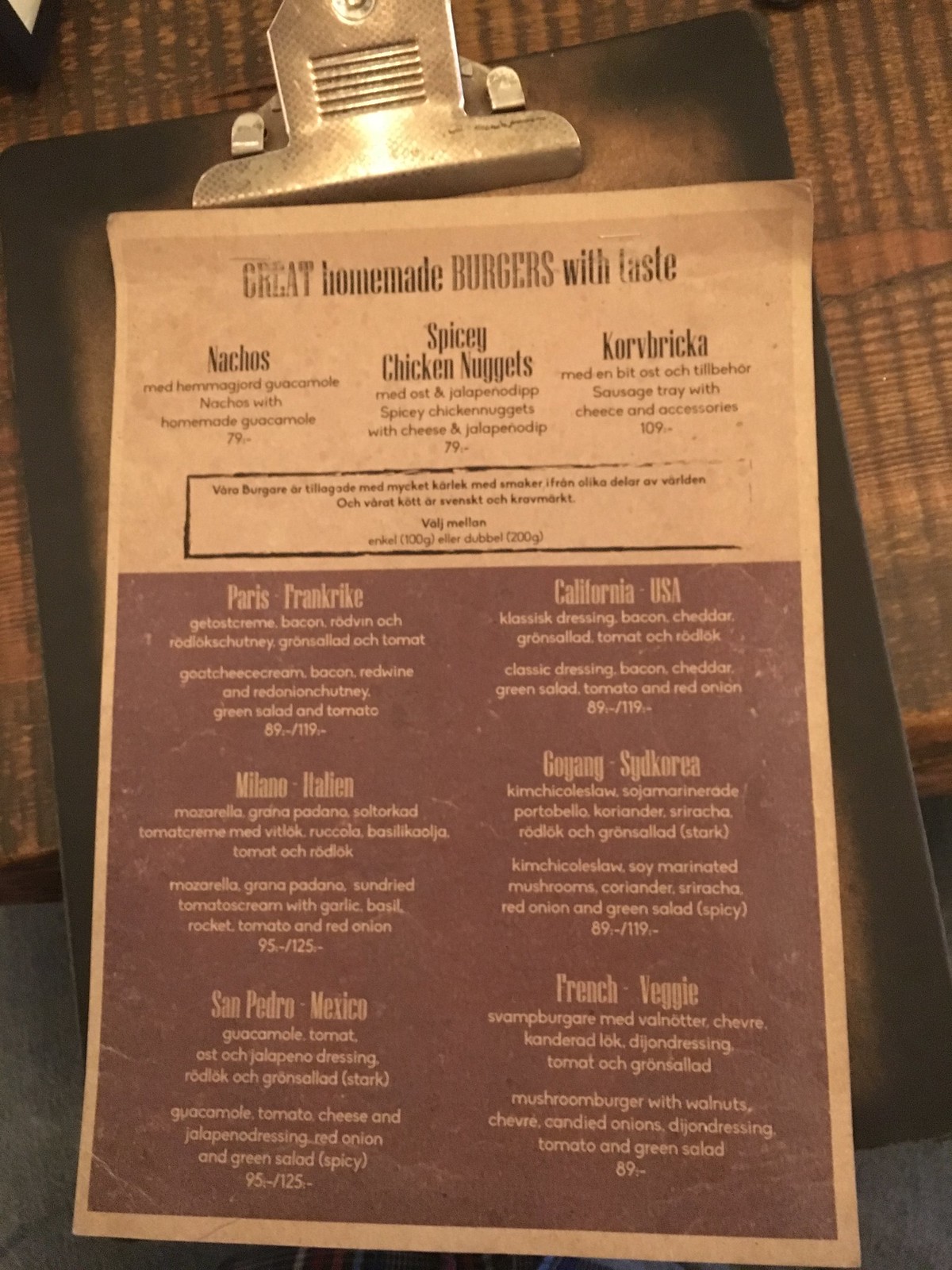The image showcases a vibrant menu from a restaurant with a distinctly Slavic flair, offering an eclectic mix of dishes from various regions around the world. Featured prominently at the top is a banner proclaiming "Great Homemade Burgers with Taste." The menu thoughtfully includes a variety of items such as nachos, spicy chicken nuggets, and a unique dish called "corvabrica," a flavorful sausage stuffed with cheese. Each dish is accompanied by a label under the "accessories" section, indicating additional condiments and sides available. Highlighted regions contributing to this diverse culinary lineup include Paris, California, Milan, Goyang, France, and Mexico, capturing a global essence while maintaining cohesive, casual dining options. This menu illustrates the restaurant's commitment to offering a rich array of international flavors, fused with the familiar comfort of homemade meals.